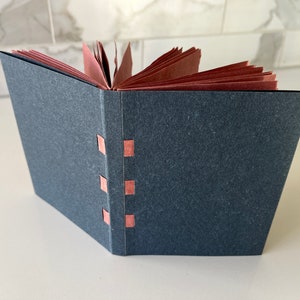The image captures a close-up of an open notebook or possibly a folder, centrally positioned on what appears to be a smooth, light-colored surface, likely a table or countertop. The notebook, with its covers in a dark grayish or bluish hue, is oriented such that its middle binding is just left of center. From this central binding, one side extends to the left and away from the viewer, while the other side stretches straight to the right. The binding itself features three vertical, pink rectangular strips that align in a column, spaced evenly from one another. Above this binding, numerous brown pages fan out in multiple directions—left, straight ahead, right, and upward—indicating either additional folder compartments or simply pages. These fanned pages are juxtaposed beneath a background that resembles a white tile or marble-patterned wall with gray streaks. The photo, taken indoors, emphasizes the stark contrast between the notebook's dark cover and the light, reflective surface it rests upon.